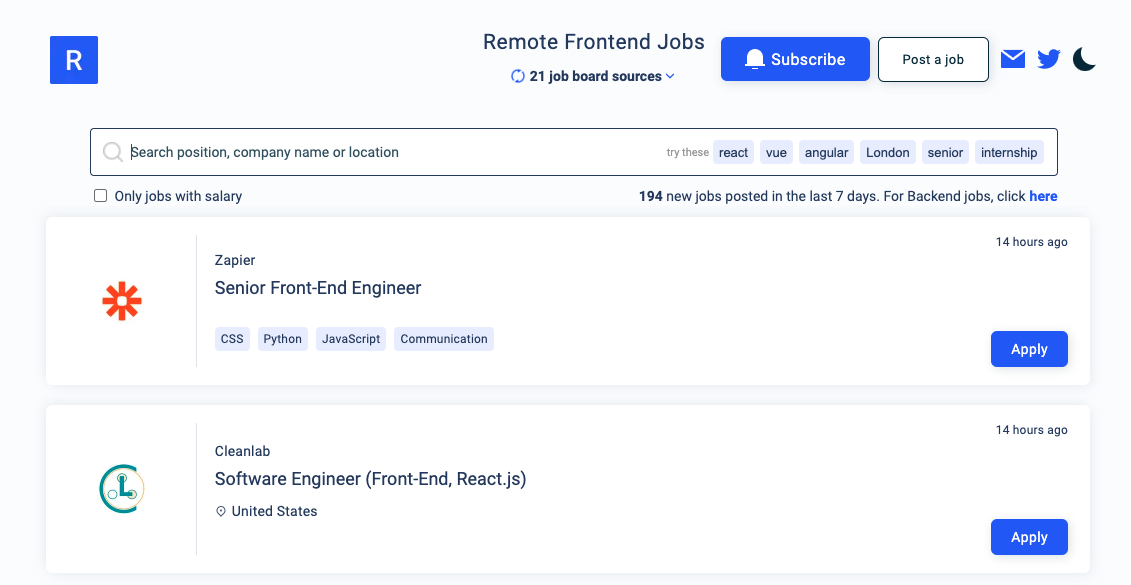The image appears to be a screenshot of a web page dedicated to remote front end job listings. In the top left corner, there's a blue box containing a white letter "R". Centered at the top of the page, bold text reads “Remote Front End Jobs.” Directly below this header, it mentions “21 job board sources.” On the right side, there is a blue button labeled "Subscribe" in white letters accompanied by a white bell icon. Adjacent to this is an option to "Post a Job", followed by icons representing an envelope, a blue bird for Twitter, and a black moon.

Beneath this section lies a search bar featuring a microphone and a magnifying glass icon, with a prompt that reads "Search position, company name, or location." To the right of the search bar, there are clickable tags labeled: "Try these: React, Vue, Angular, London, Senior, Internship."

Under the search bar, there is a checkbox option that reads "Only jobs with salary." Adjacent to it, text indicates "194 new jobs posted in the last seven days," alongside a link for "back end jobs."

The first job listing features an orange star-shaped icon and the title "Zapier Senior Front End Engineer." The job summary mentions CSS, Python, JavaScript, and communication skills, likely referring to required qualifications. To the right, a blue "Apply" button is visible, with the posting time indicated as "14 hours ago."

The second listing is for "Clean Lab, Software Engineer, Front End React.js in the United States." Similarly, it includes a blue "Apply" button and indicates the post was uploaded "14 hours ago."